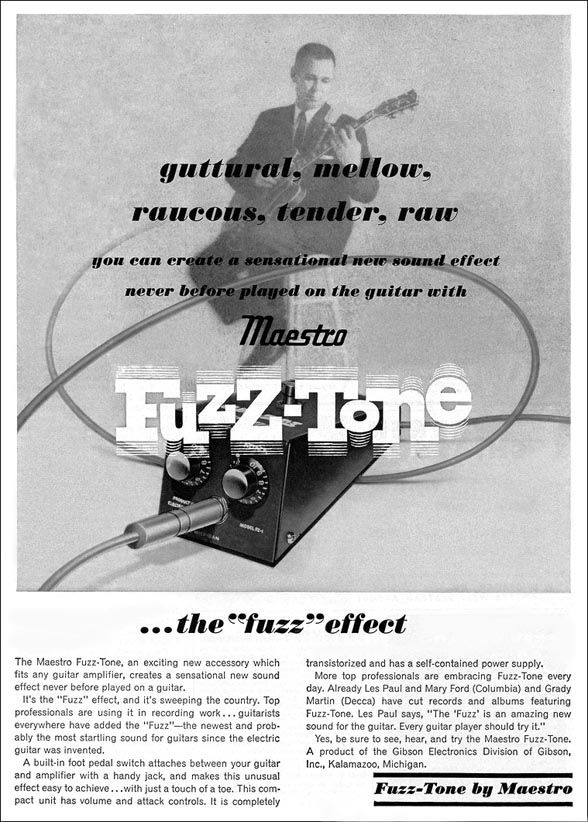The vintage ad for the Maestro Fuzz-Tone showcases a man dressed in a suit, seated on a white stool, intensely focused on his electric guitar as he prepares to strum. Above him, the bold words "guttural, mellow, raucous, tender, raw" capture the versatile tones that the Fuzz-Tone can produce. The highlighted text informs potential buyers that they can create sensational new sound effects never before achieved on a guitar with the Maestro Fuzz-Tone.

The title "Maestro Fuzz-Tone" is featured prominently in a unique font, where each letter vibrates with an electrifying effect. Below this, a detailed description explains that this innovative accessory fits any guitar amplifier to generate the groundbreaking "fuzz" effect sweeping the nation. It mentions that top professionals, including Les Paul and Mary Ford from Columbia, and Grady Martin from Decca, have already used it in their recordings. Les Paul himself endorses the Fuzz-Tone, calling it an "amazing new sound" that every guitarist should try.

The ad further describes the Fuzz-Tone's features, such as a built-in foot pedal switch that easily connects between the guitar and the amplifier, volume and attack controls, and a self-contained power supply. Overall, the Maestro Fuzz-Tone promises an unprecedented addition to the musician's toolkit, emphasizing its rising popularity and professional endorsement as a must-have innovation for electric guitarists. At the bottom right, the ad is signed off with "Fuzz Tone by Maestro," cementing its branding.